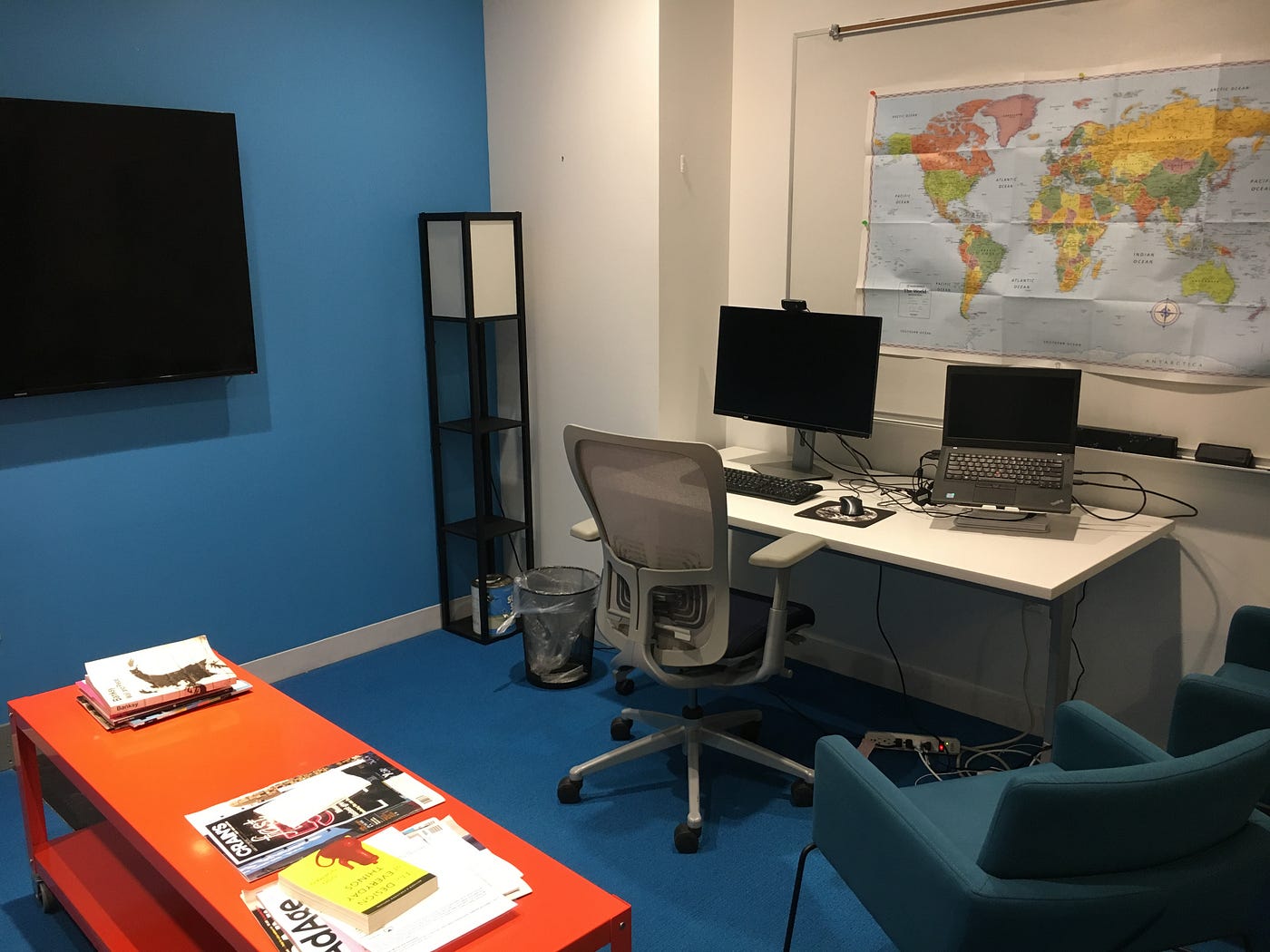The image portrays a well-organized office space. On the left side of the room, a deep blue wall is adorned with a flat-screen TV or computer screen, displayed as solid black. Adjacent is a shelving unit with a pull-string light on the top shelf. The room's focal point is dominated by a white desk positioned against a cream-colored wall, which features a map of the world pinned to a whiteboard. The map appears wrinkled, indicative of its recent unpacking. The desk hosts two computer monitors—one connected to a docking station with a laptop, a separate keyboard, and a mouse. Below the desk, cables are scattered around a modem. A sleek gray office chair with wheels sits in front of the desk.

On the floor, a low-pile, royal blue carpet adds to the room's cozy ambiance. In the lower right corner, two contemporary blue chairs provide additional seating, while a bright red shelf unit behind the desk showcases neatly stacked magazines. An orange coffee table in the lower left corner holds white and yellow magazines, offering a pop of color to the decor. The blend of royal blue, cream, and modern furnishings gives the space a professional yet vibrant aesthetic.